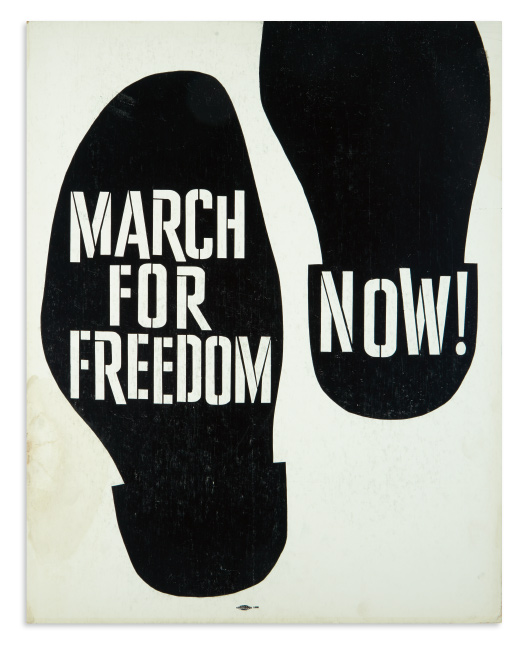The image is a vintage black and white drawing on paper that has become dingy and yellowed over time, with brownish stains, especially noticeable in the left-hand corner. It depicts two shoe prints, each showing the bottom of a shoe with bold white lettering, using a military-like block font. The left shoe print, positioned slightly lower than the right, has the words "March for Freedom" prominently displayed across the sole. The right shoe print shows only the heel, with "Now!" written emphatically. There is a black marking at the very bottom of the image, possibly the creator's signature, although it is illegible. The background is plain, with no additional elements or colors, emphasizing the stark contrast between the faded paper and the black shoe prints. This image likely served as an old advertisement or poster for a protest emphasizing immediate action for freedom.